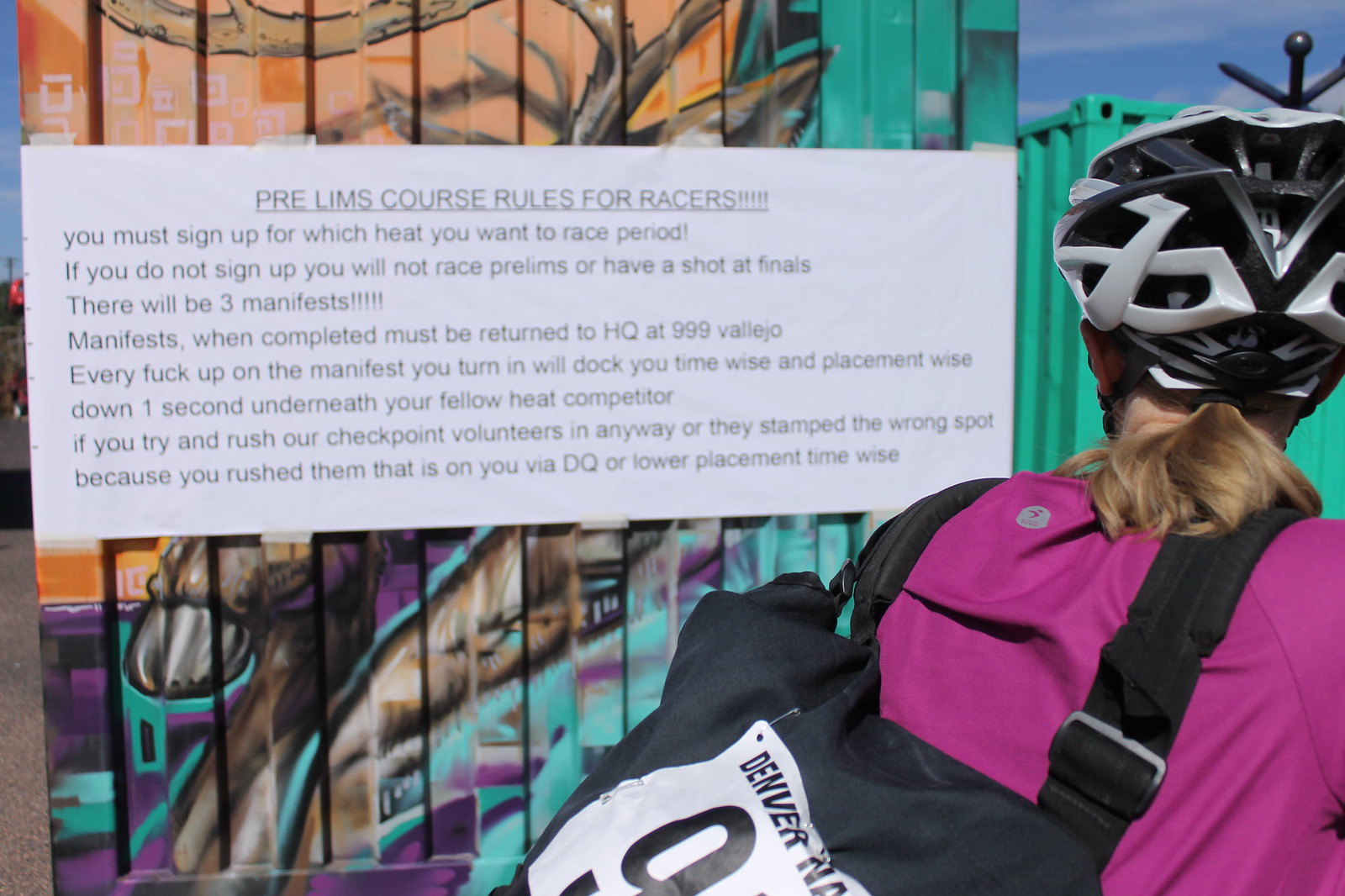The image is a daytime outdoor photograph featuring a blonde woman, wearing a black and white helmet and a purple-pink shirt, riding a bicycle. She is facing away from the camera, revealing her hair streaming out from under the helmet and not showing her face. On her back, she has a black backpack which sports a white label pinned onto it, displaying the number "9" along with the word "Denver."

She is looking at a large, rectangular white sign mounted on a fence, possibly part of a metal shipping container with graffiti that features various colors, including green and orange, and depicts what seems to be part of a tree trunk along with other objects. The sign itself is covered in black text and reads:

"PRELIMS COURSE RULES FOR RACERS!
You must sign up for which heat you want to race, period. If you do not sign up, you will not race prelims or have a shot at finals. There will be three manifests. Manifests when completed must be returned to HQ at 999 Vallejo. Any mistake on the manifest you turn in will dock you time-wise and placement-wise, down one second underneath your fellow heat competitor. If you try and rush our checkpoint volunteers in any way or they stamp the wrong spot because you rushed them, that is on you via DQ or lower placement time-wise."

The fence and the container add an urban feel to the setting, and the top right corner of the image reveals a clear, blue sky, enhancing the photograph's outdoor ambiance.